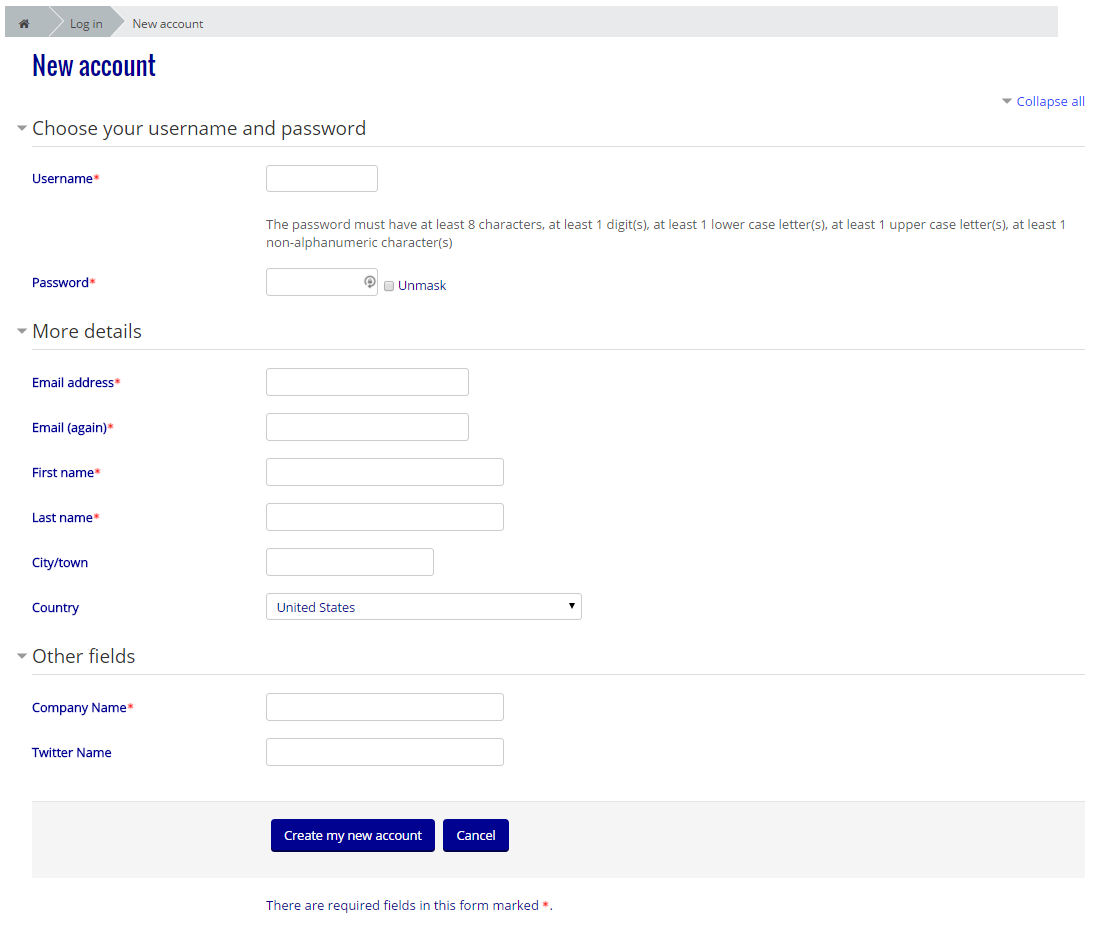The image depicts a "Create New Account" page for an unspecified website. The page has a clean, white background with a combination of black and blue text for emphasis. Users are required to fill in various fields including "Username," "Password," "Email," "Confirm Email," "First Name," "Last Name," "Company Name," and optionally "City," "Country," and "Twitter Name." The instructions for creating a password, prominently located above the password field, specify that it must be at least eight characters long and include at least one digit, one lowercase letter, one uppercase letter, and one non-alphanumeric character such as an exclamation point. At the bottom of the form, users have the options to either "Create My Account" using a large blue button or "Cancel" the process.